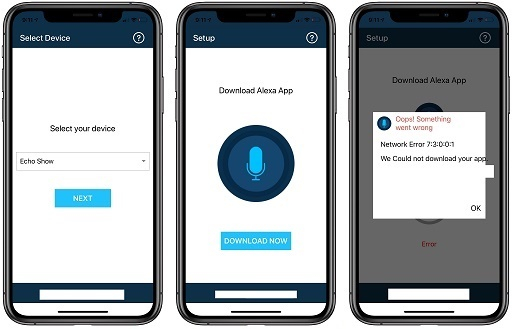The image features a side-by-side comparison of three smartphone screens, each displaying a different stage of the setup process for a device management application, likely on an iPhone.

1. **First Screen (Left):** The top left corner has a blue icon with a white text that reads "Select Device". Next to it is a white circle containing a question mark. Below this, occupying the top eighth of the screen, is a white banner with the black text "Select your device". Underneath this banner is a dropdown menu where "Echo Show" is selected. At the bottom, there's a blue button with the label "Next" in white text.

2. **Second Screen (Middle):** The layout is similar, but instead of the "Select your device" dropdown, the center of the screen displays the text "Download Alexa App" in black. Below this, prominently featured, is a large blue microphone icon. At the bottom of the screen is a blue button reading "Download Now" in white text.

3. **Third Screen (Right):** This screen appears to show an overlay warning message above the second screen's content. The warning is displayed with a red banner stating "Oops, something went wrong". Below this, black text reads "Network Error 7:3:0:0:1". The message further clarifies with "We could not download your app". The only interactive element on this screen is a button labeled "Okay" at the bottom.

The image as a whole illustrates the flow of actions disrupted by a network error during the device setup or application download process on these smartphones.